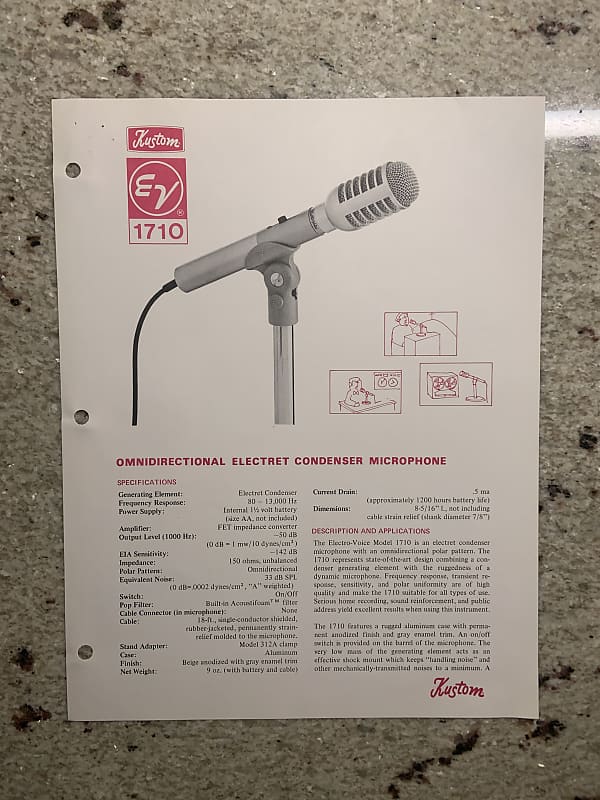The image showcases an instruction manual for a Custom EV 1710 omnidirectional electric condenser microphone. The manual is printed on a piece of white paper with three evenly spaced holes along the left side, indicating it was once part of a three-ring binder. The paper, set against a glossy stone table that reflects light, features a red box containing the model number "EV 1710" and a Custom logo, with cursive text at the bottom right spelling "Kustom." In the top middle, there is an image of the gray microphone mounted on a stand, with a wire trailing off. The textual content includes specifications for the microphone, descriptions of the generating element, and its applications, along with three cartoons illustrating use cases. The writing on the manual is primarily in black, providing detailed setup instructions and specifications.